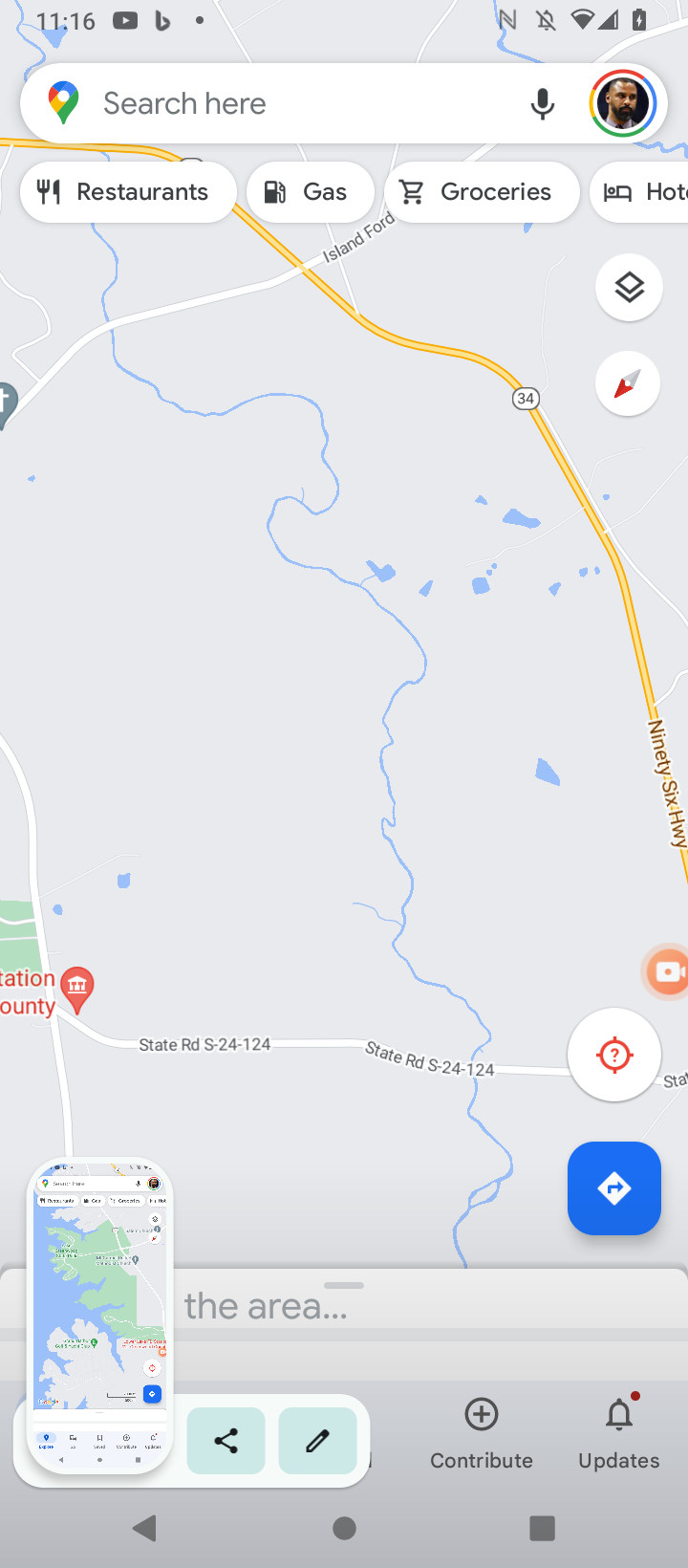This image showcases a screenshot from the Google Maps app, displayed as it would appear on a smartphone. The upper section of the screen features navigational information, depicting an orange-highlighted route that appears to involve travel along a parkway and a highway, possibly labeled as Route 34. The surrounding area on the map looks relatively sparse, with minimal geographical details or landmarks aside from the mapped-out path.

At the top of the image, there are options for users to search for nearby points of interest such as restaurants, gas stations, grocery stores, and popular attractions. Users can enter their desired search terms in the search bar provided.

Below the navigational map, the screen includes an inset of another map, offering additional functionalities like an update feature and a contribute feature.